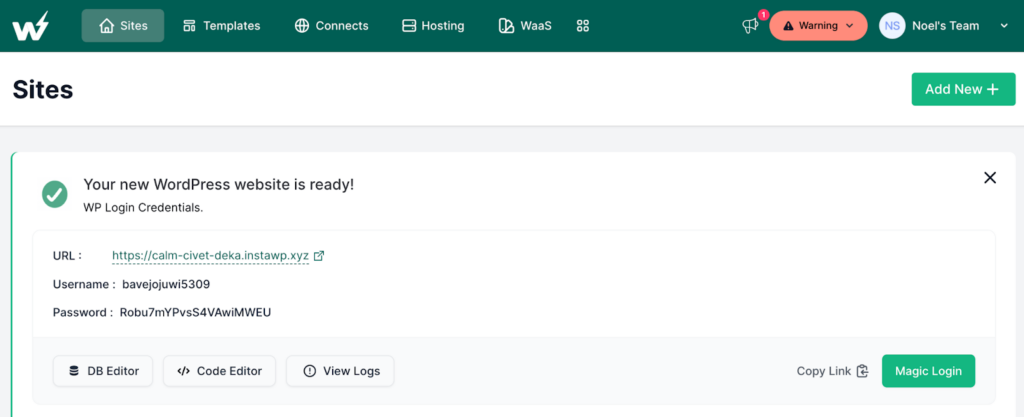In the image, the central focal point is a prominent black rectangle featuring a stylized "W" with a lightning flash at its end, followed by the terms "Sites," "Templates," "Connects," "Hosting," and "WAAS." Adjacent to this, there's a red rectangle labeled "Warning," and above that is "Noel's Team."

Below this section, a white rectangle is displayed, containing the word "Sites" on the left side and "Add New" on the right, next to a green button. To the left, there's a green circle encompassing a checkmark beside the text "Decided." The accompanying text reads "Your New WordPress Website is Ready," followed by "WP Login Credentials," and then details such as "URL," listing a website address formatted as "HTTPS://COM/CIVET/INSTAWP/X/Y/Z."

Further, it provides the "Username" as "Baba Joju W15309" and a corresponding "Password." There are additional options listed as "DB Editor," "Code Editor," and "VLogs."

On the right-hand side of the image, a black "X" icon is located next to a green button labeled "Magic Login."